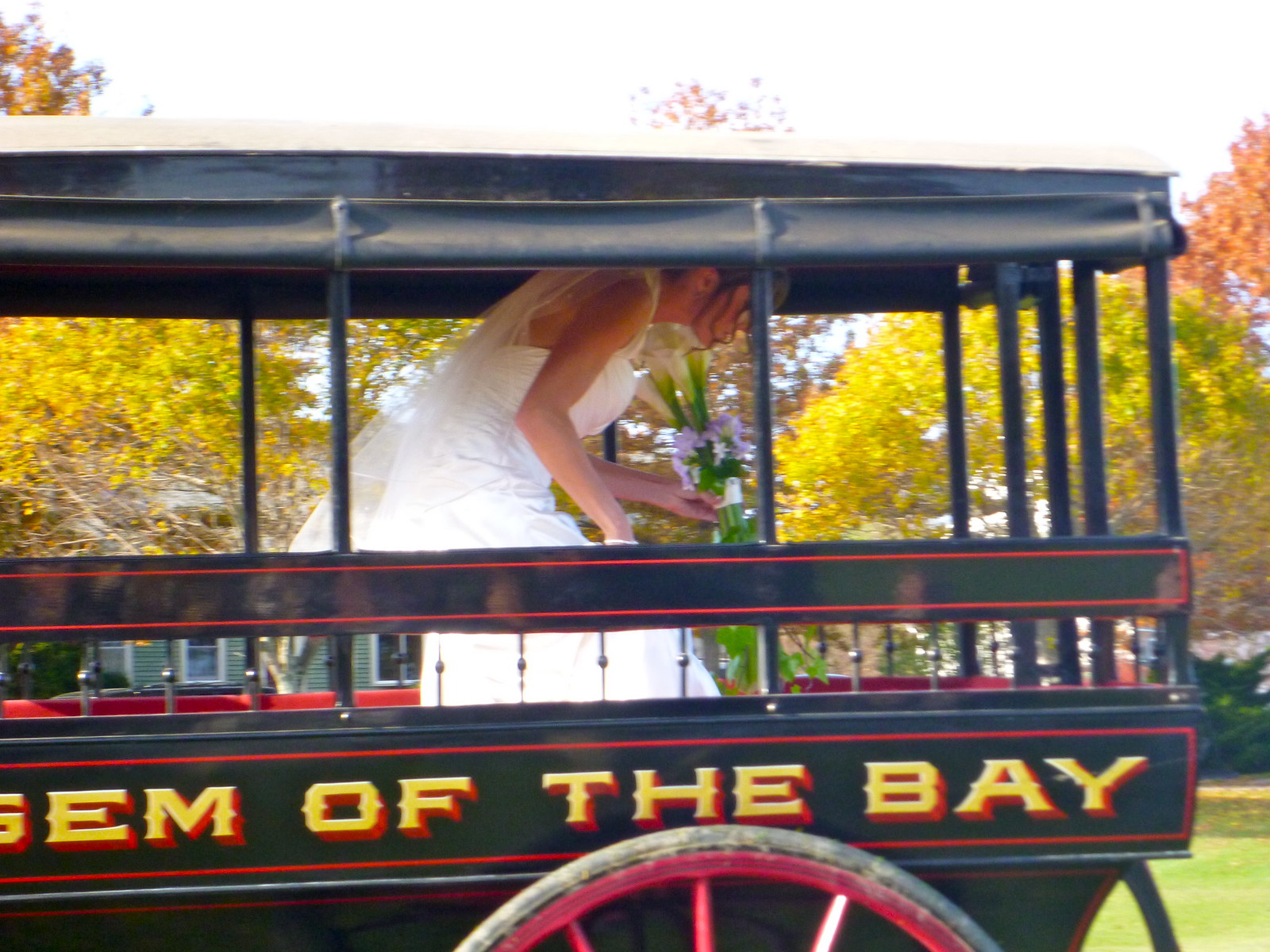In this outdoor photograph taken in a park-like setting during the early fall, a bride dressed in an elegant white wedding gown and holding a bouquet is captured as she steps out of a black carriage. The carriage, which features a roof and open sides with bench seating, has large red wheels and yellow text partially visible on its body, reading "of the bay." The bride, central to the image, appears to be mid-movement, as though she is either crouching or in the act of leaving the carriage. Surrounding her in the background are a variety of trees with leaves in shades of yellow, green, and orange, indicating the autumn season. The grass underfoot is lush and green, adding to the vibrant outdoor atmosphere of this charming and picturesque scene.